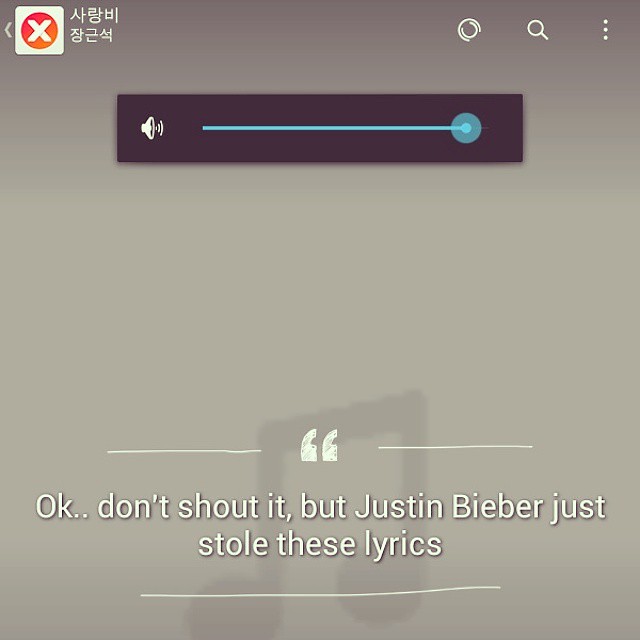This image is a detailed screenshot of a music app on a phone with a predominantly gray background. At the top left corner, there's a left-pointing arrow followed by a square white box enclosing a red circle with an "X" symbol inside. To the right of this, there's text in a Korean or Chinese script. Further right, there is a magnifying glass icon for search functionality and a three-dot menu icon for additional options. Beneath this, there is a slim black volume bar with a white speaker icon on the left emitting sound waves, and a blue slider pushed all the way to the right, indicating the volume is at its maximum. Below the volume bar, the screen continues with a gray background displaying white text that reads, "Okay, don't shout it, but Justin Bieber just stole these lyrics."